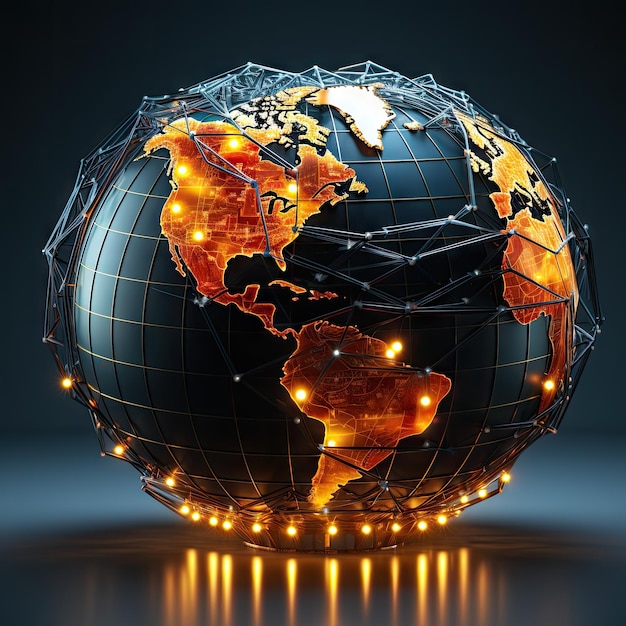The image depicts a computer-generated globe with dark blue oceans highlighted by latitude and longitude grid lines, without a detailed depiction of water. The continents, shown in a dark orange or yellow hue, appear slightly elevated above the surface, emphasizing a plastic-like texture. Scattered across these continents are bright, small lights, possibly representing major cities or technological hubs. Additionally, metal-like lines, resembling steel wires or a satellite framework, crisscross the globe, indicating possible routes or networks. Reflections of the glowing lights can be seen on the smooth blue surface on which the globe rests. The image features a gradient background that transitions from dark at the top to lighter towards the bottom, enhancing the overall high-tech and abstract aesthetic.